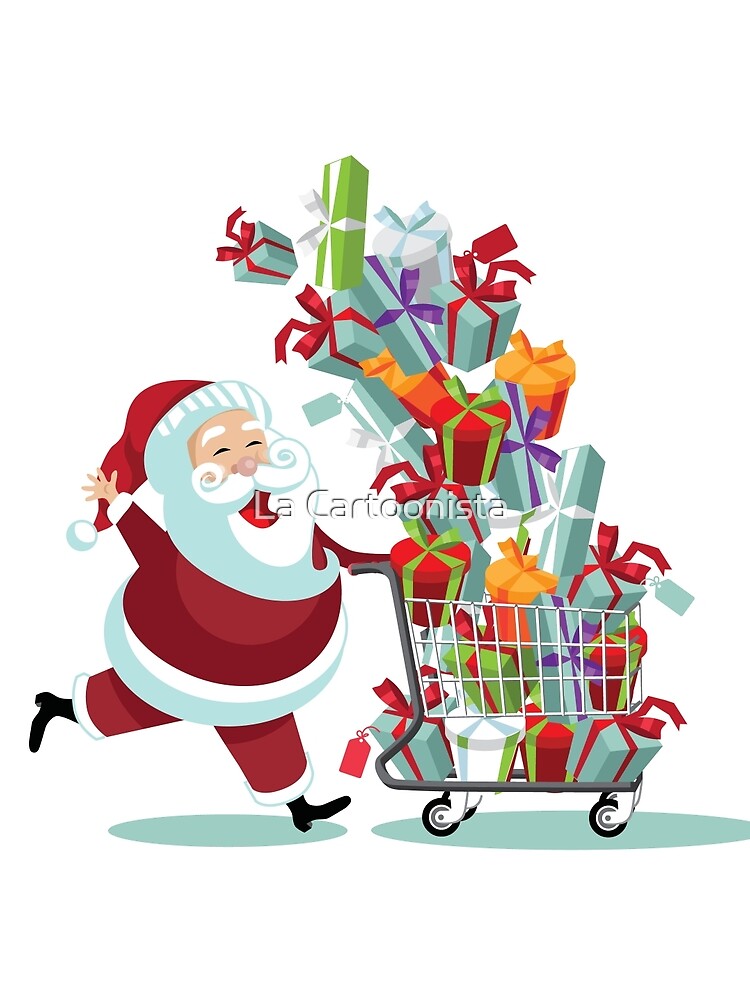A vibrant and cheerful cartoon of Santa Claus is depicted, dressed in his iconic red suit adorned with white fur trimmings and a matching red cap featuring a white brim and a fluffy white pom-pom. His black shoes are visible as he pushes a supermarket-style shopping cart overflowing with brightly wrapped presents. The gifts, in an array of colors including reds, blues, yellows, greens, oranges, and purples, are stacked precariously high, extending well above Santa's head. He is smiling broadly and waving with his right hand, exuding joy and warmth. The image includes the detail of green oblong shadows beneath Santa and the cart, adding depth. In the middle of the drawing, the words "La Cartoonista" are inscribed, adding a signature touch to the festive scene.